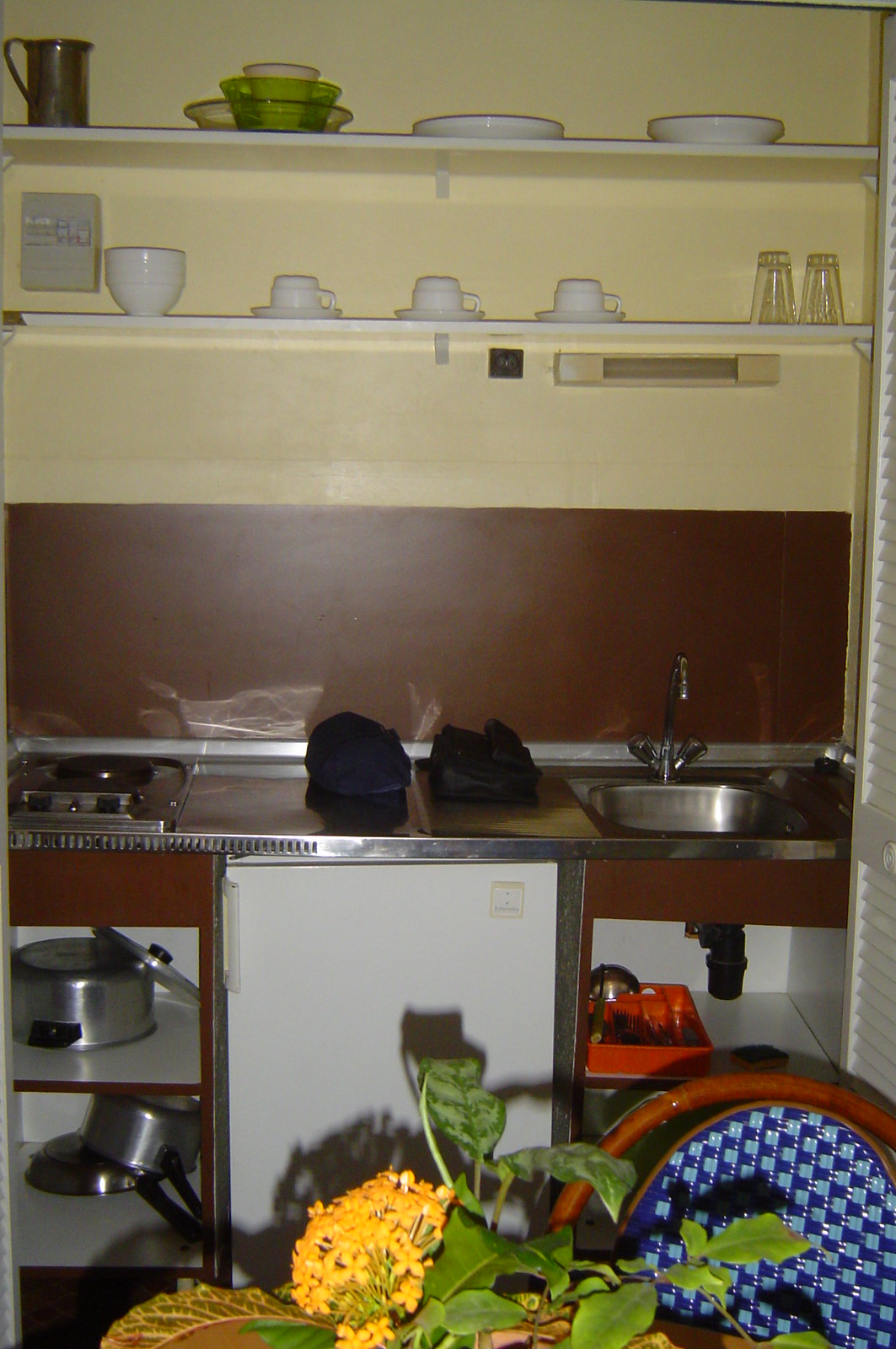This vertically aligned, portrait-style photograph captures the essence of an old-style kitchen, shot in low lighting. The kitchen features a beige upper wall section, with two white shelves stacked with various dishware. The top shelf is home to a collection of green dishes and white bowls with gold rims, while the bottom shelf holds an assortment of white dishes, coffee mugs, saucers placed upside down, and drinking glasses. Beneath this, a darker brown wall section frames a stainless steel sink on the right, equipped with a faucet featuring two levers. To the left of the sink, a black object rests on the stainless steel countertop, adjacent to what appears to be the burners of a stove. The lower section of the image reveals open white shelves holding pots, pans, and a dorm-style small refrigerator. Additional storage on these shelves includes a red cutlery holder. At the very bottom of the image, shadows emphasize the low lighting, partially obscuring a yellow flower with green leaves. In the lower right-hand corner, the curved top of a brown kitchen chair with a blue checked seat back is visible, hinting at a dining area just in front of the photographer.